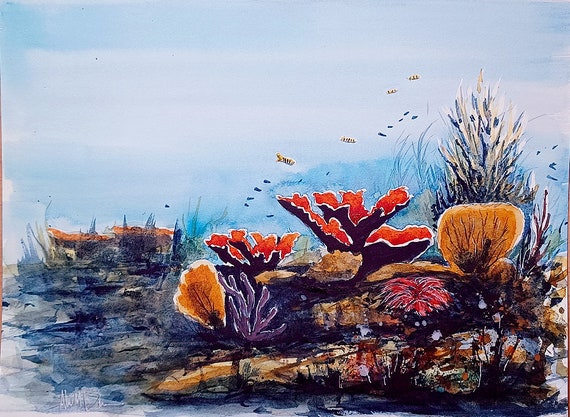This image is a detailed, watercolor painting depicting an underwater coral reef scene. The sky-blue water merges seamlessly with horizontal clouds, creating a smooth, dreamlike appearance that almost makes the scene look as if it could be above water. In the foreground, various species of coral in vivid hues of red, orange, yellow, and purple dominate the lower half of the painting, particularly concentrated at the bottom center and extending towards the right. Among the corals are red and purple sponges, interspersed with sea cucumbers and vibrant green and orange sea anemones.

Clusters of fish, including yellow ones with white stripes and several distant blue ones, swim harmoniously above the colorful reef. Some fish are harder to identify due to their distance, but they form distinct schools that weave through the scene, both above the corals and dispersed finely throughout the painting. The coral and sea life, detailed meticulously, establish that this scene truly captures the essence of a vibrant underwater ecosystem. With hints of sea grass peeking out and the gentle blending of colors, the overall composition of the painting beautifully portrays the symbiotic coexistence of marine life within this coral reef, giving viewers a serene glimpse into the underwater world.